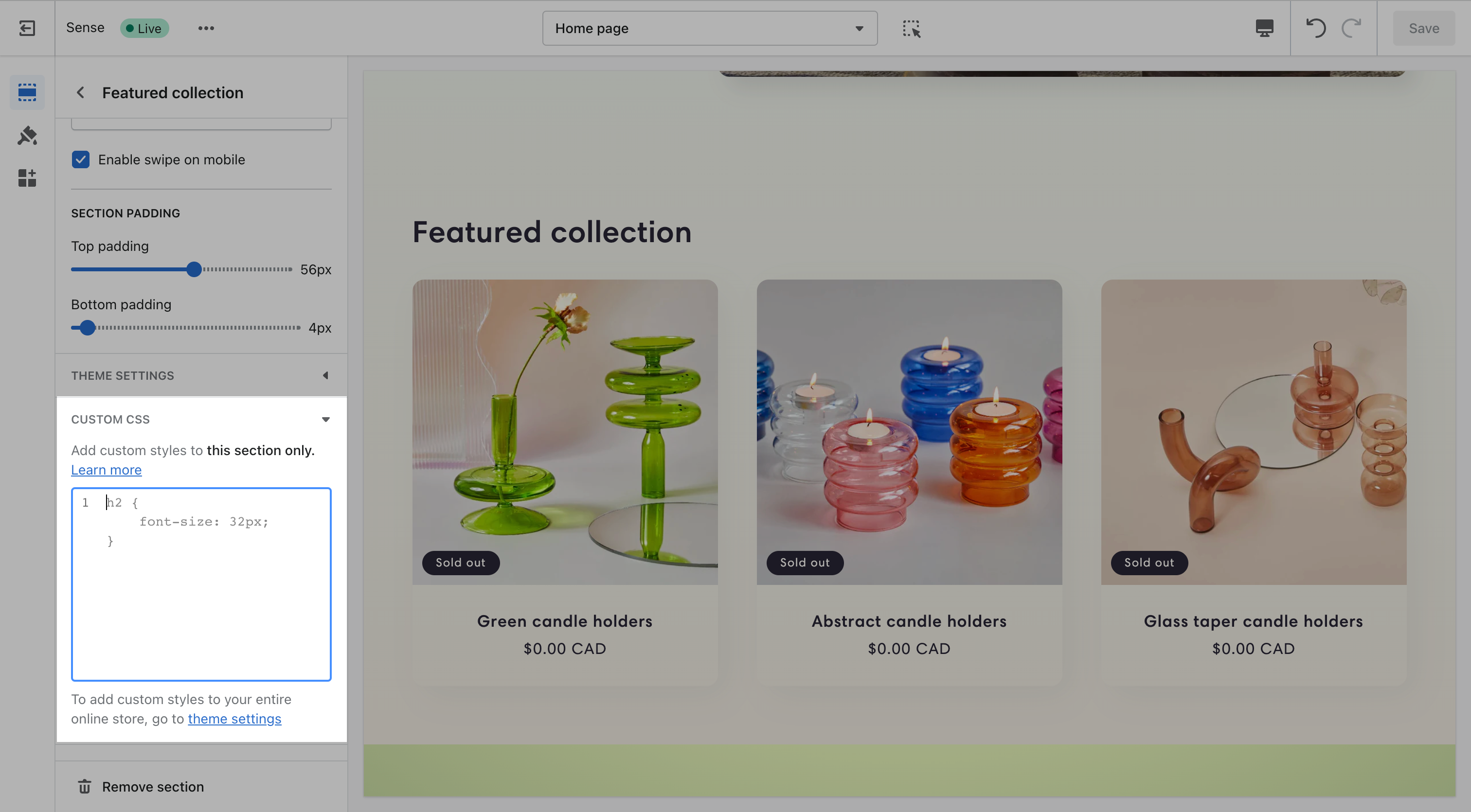This detailed screenshot captures the interface of a web-based application, likely focused on e-commerce or digital content management. 

**Top Bar:**
- The top left corner displays the word "sense" alongside a green "live" indicator.
- Centered at the top is the label "homepage."

**Main Content:**
- On the right side of the screen, under a section titled "Featured Collection," three distinct candle holder images are displayed.

**Candle Holder Descriptions:**
1. **Green Candle Holders**:
   - Features a set of green candle holders.
   - They have a flat base with a circular bottom and a skinny stem rising up.
   - A flower decorates the holders.
   - Labeled as "Green Candle Holders," priced at 0 CAD, and marked "Sold Out."

2. **Abstract Candle Holders**:
   - Displays a unique design featuring white, pink, blue, and orange candle holders.
   - These holders appear to be constructed from three clear glass rings.
   - Labeled as "Abstract Candle Holders," also priced at 0 CAD and marked "Sold Out."

3. **Glass Taper Candle Holders**:
   - Showcases yellowish candle holders made from different shapes.
   - One holder resembles a stack of discs, while another appears to be a twisted line.
   - Labeled as "Glass Taper Candle Holders," again priced at 0 CAD and marked "Sold Out."

**Additional Interface Elements:**
- On the left side of the screen is a pop-up labeled "Custom CSS."
    - This pop-up allows the addition of custom styles specific to this section.
    - It includes a large blue textbox for inputting custom CSS code.

This comprehensive and precise description covers all visible elements and their details in the provided screenshot.